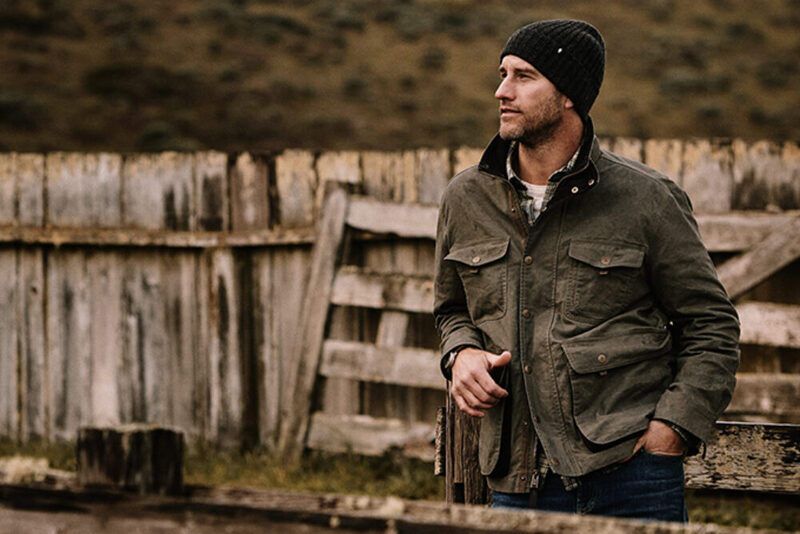The image depicts a young man in his late 20s or early 30s standing outside against a weathered wooden fence. He is positioned slightly to the right and gazes towards the left. The man is wearing a dark olive green, light brown jacket with four pockets, snapped closed over a flannel shirt and a white t-shirt. He has a thin black mustache and beard, and wears a black knit cap covering his head. His left hand is tucked into the pocket of his blue jeans, while his right hand hangs by his side. 

Behind him, the wooden fence, visibly old with some missing planks, stretches across the background. The fence has vertical boards in a horizontal row, displaying a faded mix of brown, gray, and black hues. A gate leans against the fence, contributing to its decrepit appearance. Further back, one can make out a somewhat blurry hill, dotted with lighter and darker green sections of grass and shrubs. In the foreground, the ground is covered with grass and scattered weeds. To the far right of the image, the beginning of another fence, which gets cut off, is also visible.